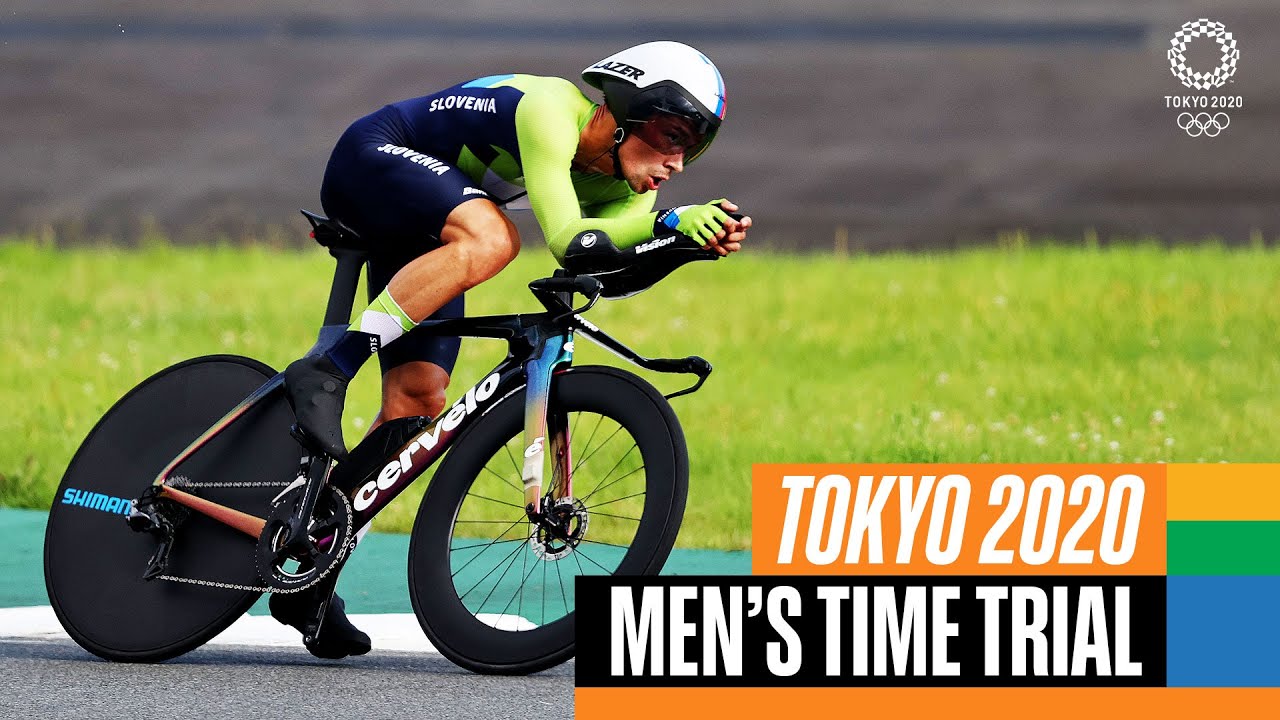The image is a detailed advertisement poster for the Tokyo 2020 men's time trial. Prominently displayed on the top right corner is the Tokyo 2020 Olympics logo. Below this, large bold text reads "Tokyo 2020 Men's Time Trial" against an orange and black background. Central to the poster is a dynamic depiction of a Slovenian cyclist, garbed in a tight, colorful leotard featuring shades of blue and green with "Slovenia" emblazoned on the side. The cyclist is leaning aggressively forward, showcasing his aerodynamic stance. He wears a white, futuristic helmet with a black visor covering his eyes, and brown goggles underneath. His bike is notably high-tech, featuring a fully black, disc-shaped rear wheel and a spoked front wheel. The frame bears the name "Sir Velo." The cyclist's outfit includes long sleeves and navy, tight-fitting shorts, with one distinctly green glove, and cyclist shoes that extend nearly to his crew socks. In the background, the scene is set along a road lined with light green grass, leading into a stadium nestled amid gray stands. The entire composition vividly captures the intensity and futuristic vibe of the high-stakes Olympic race.